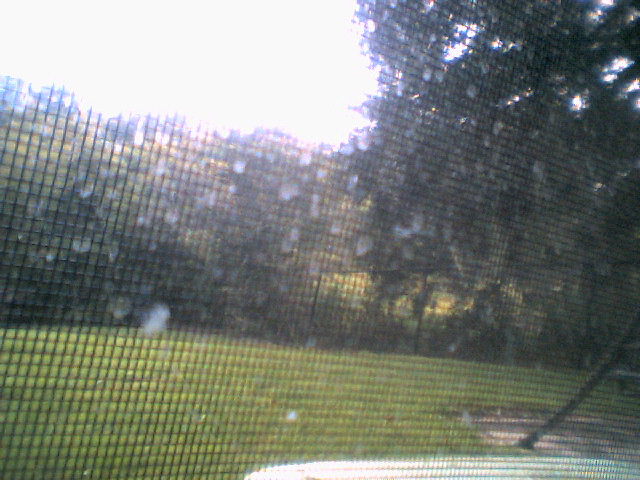A detailed caption for this image can be:

---

A close-up photograph taken through a wire frame screen reveals the intricate network of thin metal wires in sharp focus. The background, blurred by the camera’s focus on the screen, hints at a serene outdoor setting. A well-maintained lawn of short grass extends across the scene, bordered by various plants, bushes, and possibly trees. The foliage is indistinct, blending into a blur of greenery due to the camera's depth of field. In the bottom right corner, a curved tree trunk juts into the frame, extending diagonally towards the top left of the image. The brightness of the daylight is overwhelming towards the upper left, washing out details and obscuring the sky. The image is sprinkled with dust particles or light specks, creating a bokeh effect that adds a dreamy, atmospheric quality.

---

This caption offers a vivid and detailed description that captures the nuances and elements of the image.